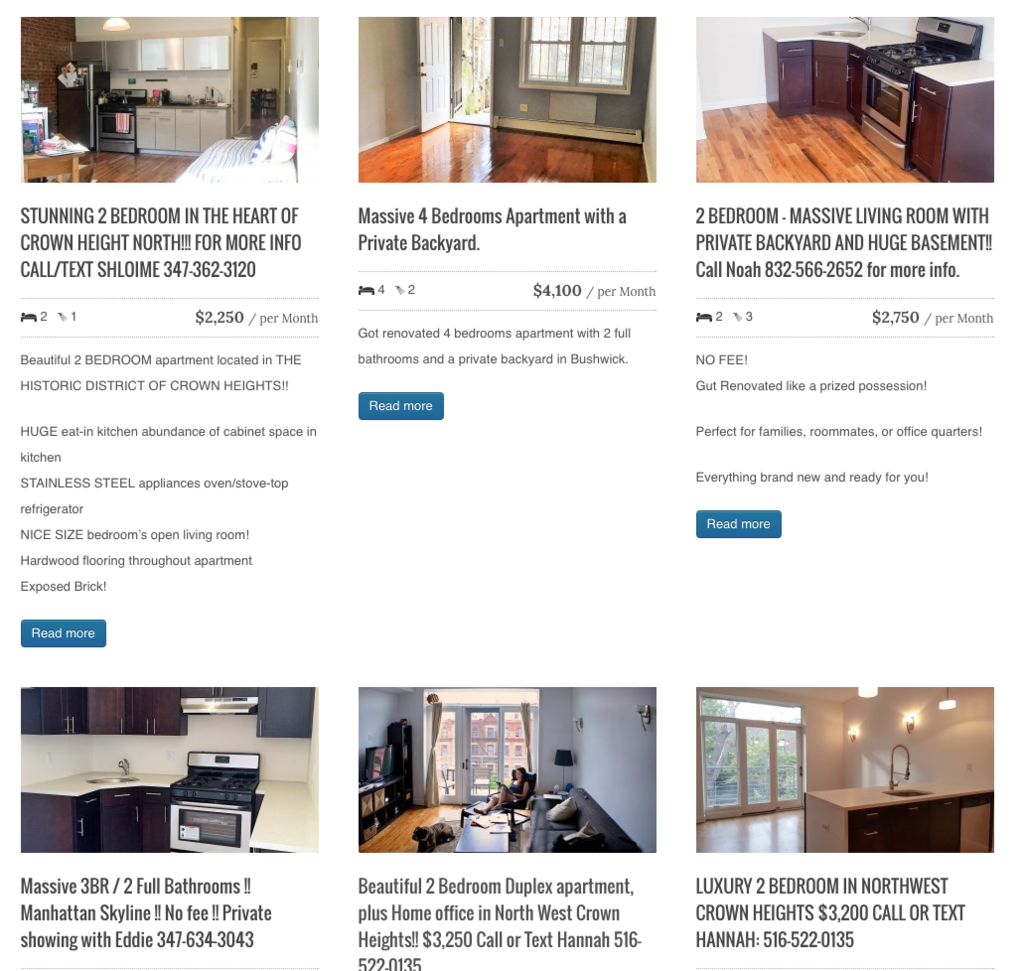**Detailed Descriptive Caption:**

This image is a screenshot of a website for renting apartments, showcasing multiple listings. 

1. **First Listing:** 
   - **Image Description:** The first listing features a cozy and stylish kitchen area accompanied by a white couch with decorative pillows. The kitchen includes a refrigerator, an oven, several cabinets, and a small dining table.
   - **Listing Details:** 
     - Property: Stunning two-bedroom apartment
     - Location: Heart of Crown Heights North
     - Contact Information: For more details, reach out to Shlomi at 347-362-3120 via call or text.
     - Features: This beautiful two-bedroom residence includes one bathroom and rents for $2,250 per month. The apartment boasts a huge eat-in kitchen with an abundance of cabinet space and stainless steel appliances such as an oven, stovetop, and refrigerator. The bedrooms are spacious, and the open living room features hardwood floors throughout and exposed brick accents.
   - **Call to Action:** There is a blue button with white text that reads, "Read More."

2. **Second Listing:** 
   - **Image Description:** The second listing shows an inviting front door with a window, opening to a living space with grey-painted walls and shiny wooden floors.
   - **Listing Details:** 
     - Property: Massive four-bedroom apartment with a private backyard
     - Location: Bushwick
     - Features: This newly renovated apartment has four bedrooms and two full bathrooms, with the added luxury of a private backyard. The asking rent is $4,100 per month.
   - **Call to Action:** A "Read More" button is also present for this listing.
   
3. **Third Listing:** 
   - **Image Description:** A separate entry shows a spacious two-bedroom apartment with an extensive living room area.
   - **Note:** Details for this specific listing were not fully provided in the excerpt.

Each listing provides essential information about the properties, highlighting key features and amenities, along with contact and further action options for potential renters.